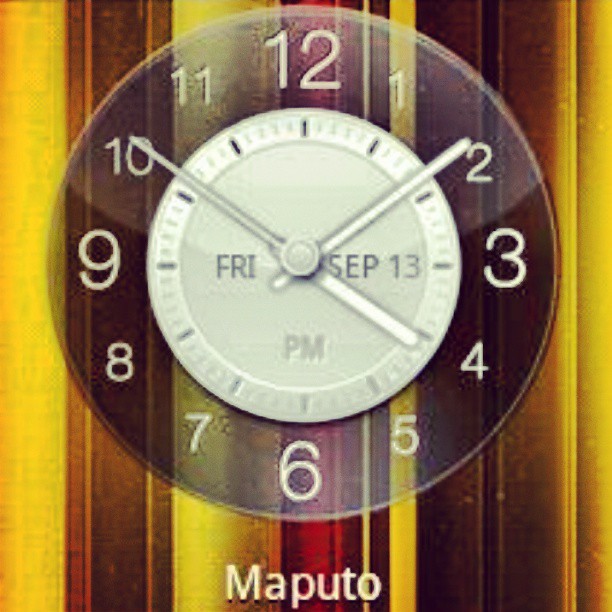This image depicts a digitally created-rendering of a round, translucent clock, prominently displaying the date "FRI, SEP 13" and the time in the PM. The clock has a silver central face where the three clock hands are anchored: the minute hand points to the 2, the hour hand to the 4, and the second hand to the 10. Encircling the central face are large white numerals marking the hours, with the 12, 3, 6, and 9 depicted slightly larger than the other numbers. The background of the image consists of vertical stripes in shades of yellow, brown, and red, resembling wood paneling. At the bottom of the image, in white text, the word "Maputo" is displayed.